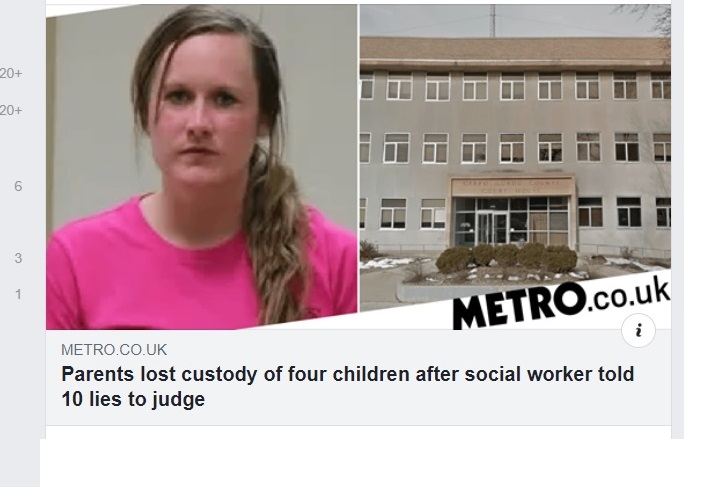This image is a screenshot from a news website, likely from metro.co.uk, featuring a clipping of a news article. In the upper left corner, there's a photo of a white woman with brown hair styled in a ponytail draped over her left shoulder. She's wearing a pink crew-neck shirt and faces the camera without a smile, reminiscent of a mug shot. Below her photo, "metro.co.uk" is written in gray letters, followed by a black-lettered article title detailing that "parents lost custody of four children after social worker told 10 lies to judge." Adjacent to her image, there's a picture of a gray building with numerous white-trimmed windows and a flat tan-brown roof. The building appears to be a courthouse, featuring a glass front and an awning. In front of the main entrance, a circular pathway surrounds a garden bed with shrubbery and gravel. Below this image, the text "METRO.CO.UK" is written in black capital letters, aligning with the website's branding. The entire presentation resembles a news report from the United Kingdom, highlighting significant legal and social issues.